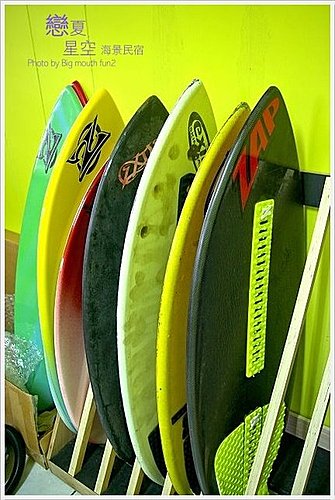The photograph showcases a vibrant lime green wall adorned with Japanese characters in the upper left-hand corner, accompanied by the English phrase "Photo by Big Mouth Fun 2" written in purple lettering. In front of this backdrop, a display rack constructed from light-colored wood with black base slots holds an array of surfboards. The stand's diagonal slats create organized spaces for the boards to be neatly stored side by side. The surfboards feature a spectrum of colors, including black, yellow, white, red, and lime green. Specifically, from left to right, the first surfboard is black with the word "Zap" in red lettering and a green base. Following that, there is a yellow surfboard, then a white one, succeeded by another black surfboard with white graffiti-like lettering. Next is a vibrant red and pink two-tone surfboard, then another yellow one, and finally a green surfboard with a yellow accent and red lettering, possibly with a red surfboard behind it. This arrangement of body boards suggests their use for beach activities, where one might run and slide in shallow waters.